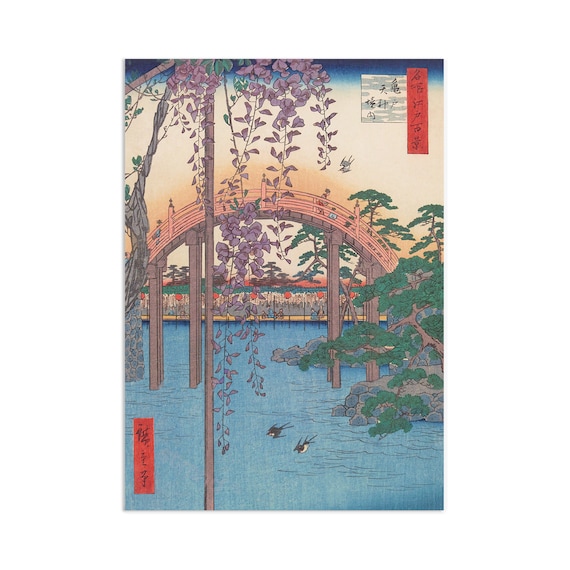This detailed and colorful illustrated print portrays a serene Japanese landscape, likely reminiscent of traditional artwork you might find in a Japanese or Chinese restaurant. Dominating the scene is a graceful, high-arching wooden bridge with railings, supported by columns on either side, though not directly in the center of the arch. The bridge arcs elegantly over a tranquil blue pond or river, where two small cranes can be seen, implying a sense of peacefulness. The water occupies the lower portion of the image, giving way to a backdrop where land is faintly visible beyond the bridge.

In the immediate foreground, cherry blossoms hang into the water, while flowering vines with purple flowers extend from the top edge of the image. A tall and narrow tree extends from the bottom edge to the top, and on the right side, a lush green tree with hanging leaves and rocks below adds depth to the composition. Among the natural beauty, a few people are visible, walking leisurely across the bridge, enhancing the scene with a human touch.

The upper right and lower left corners of the image feature vertical rows of kanji text, each on a striking red background. The upper side contains five characters, while the lower side has three. Despite the low resolution of the print, the classic Japanese aesthetic is evident, with intricate details that make the artwork visually captivating.